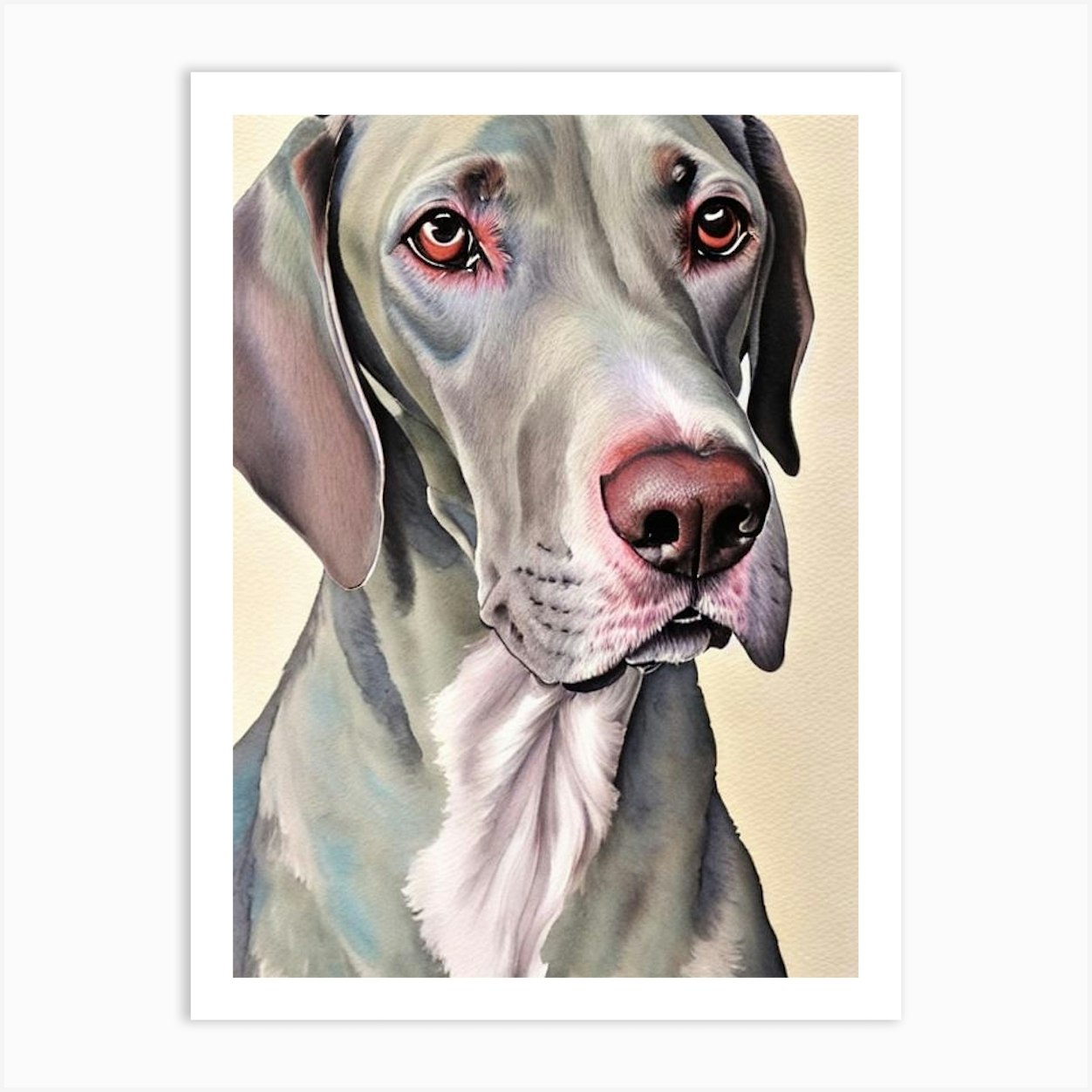This detailed illustration captures a portrait of a gray hound dog, featuring both its face and neck down to the tops of its front legs. The dog has a smooth coat with a grayish-blue hue, complemented by a distinctive white blaze on the front of its chest. Its muzzle has subtle white patches and it boasts a velvety texture. The dog's floppy, long ears are notably darker, with the right ear showcasing a darker brown or gray, and the left ear having a pinkish tone. The ears drape softly below its head, adding to its aged and dignified appearance.

The dog's nose is predominantly black with some red elements, and its snout is large, reflecting characteristics of a hunting dog. Its eyes are light red or pink, hinting at an older age, and there are brown spots above the eyes. Around the nose and muzzle, there's a soft pink coloration. 

The background is a plain, pale cream or beige tan color, highlighting the dog’s defined features. The portrait is framed in a white border, drawing attention to the finely detailed illustration.